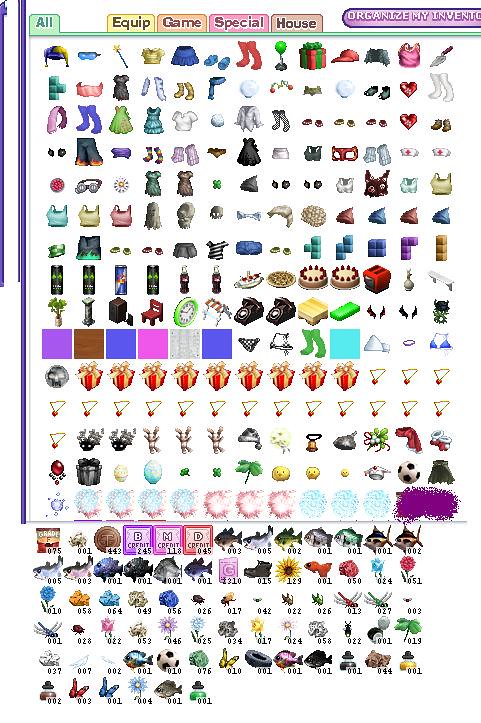This image appears to be a screenshot from a computer or mobile game, likely taken in the 2000s. The interface showcases a detailed inventory screen with hundreds of colorful icons representing various in-game items. At the top of the screen, several tabs are visible: "All," "Equip," "Game," "Special," and "House." The "All" tab is currently selected, displaying a comprehensive view of all available items.

The items include a wide array of objects such as clothing (pants, shirts, boots, glasses, necklaces, hats, socks), accessories (goggles), and other miscellaneous items like shoes, gifts, a Christmas gift box, a Red Bull can, an energy drink can, a chair, telephones, and cakes. There are also sports-related items like a soccer ball, and natural elements like flowers and various fish species (blue fish, white fish, marine fish).

In the top right corner, there is a partially visible purple button labeled "Organize My Inventory," suggesting that the user can sort and manage their items. This detailed assortment of icons strongly suggests that the screenshot is from a game that involves a significant element of item collection and organization, reminiscent of games like "The Sims."